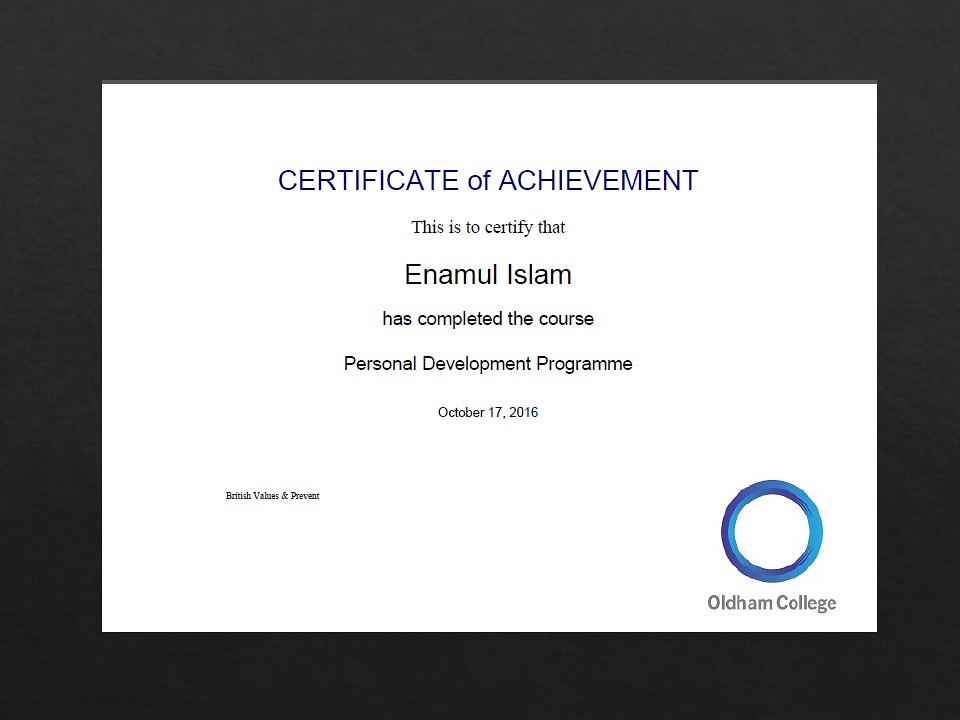The image is a horizontally-oriented rectangular Certificate of Achievement with a minimalistic design, bordered by a solid black frame. The center of the certificate features a white background with centrally aligned black text. At the top in blue, the text reads "Certificate of Achievement". Below this, in black, it states: "This is to certify that Enamul Islam has completed the course, Personal Development Program, October 17, 2016," with "Enamul Islam" in bolder black print. In the bottom left corner of the white background, there is smaller black text that reads "British Values and Prevent". On the bottom right, there's a blue circle, and beneath it, the gray text states "Oldham College".